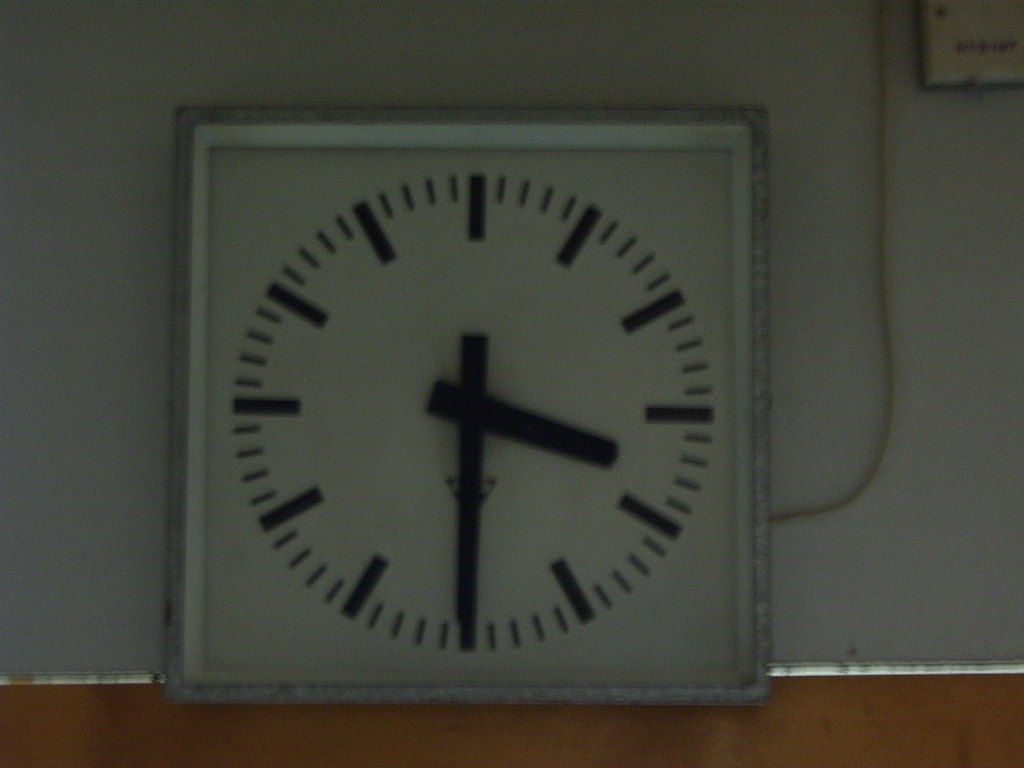The image depicts an indoor scene viewed from left to right. At the bottom of the image, there is a brown strip that could either be part of the floor or a section of the wall dividing two different areas. Above this, there's a gray section, which seems to be part of the wall. This gray wall has varying shades due to shadows being cast upon it. Emerging from the wall is a cord connected to a partially visible cream-colored box. Additionally, there is a clock mounted on the wall. The clock features a sleek steel gray rim followed by a white frame around its face, which is also white. The clock's design is minimalist, with no numbers, only thicker black lines marking the hours and shorter black lines for the minutes. The clock hands are also thick and black, adding to its modern aesthetic.